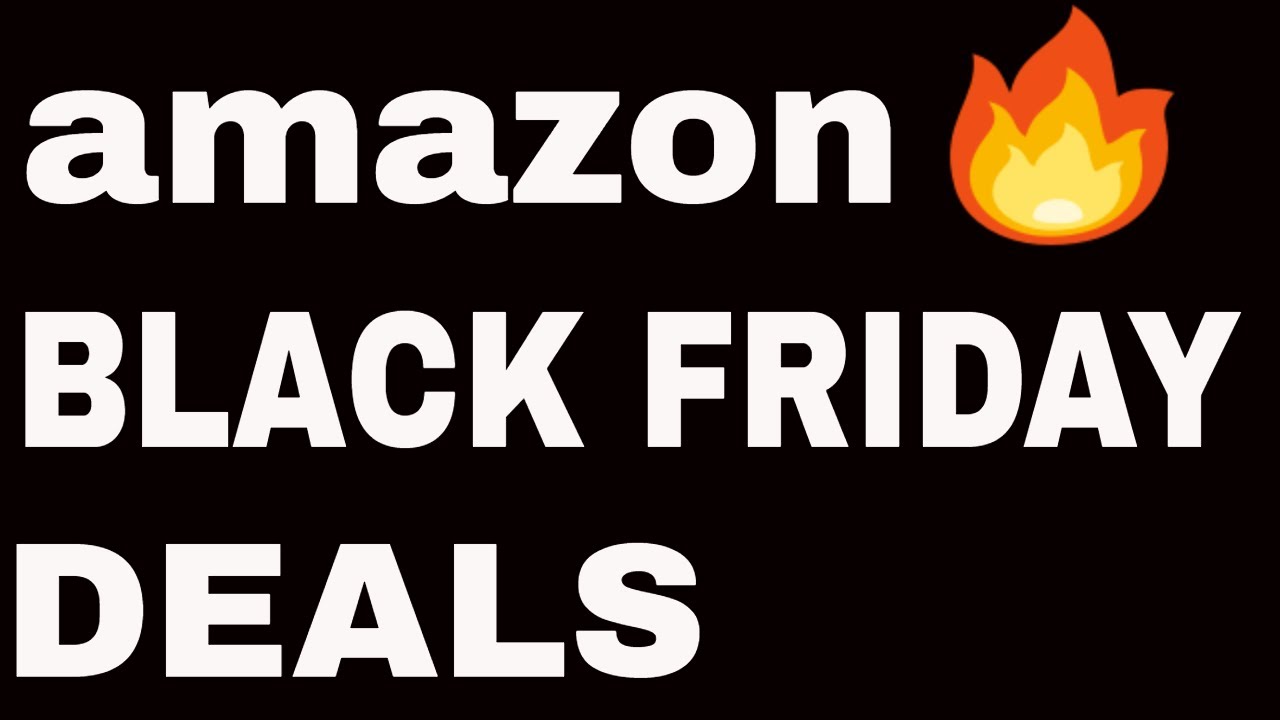This image features a striking, minimalist design set against a deep black background, which exudes a sleek and modern aesthetic. Prominently displayed in bold, white, uppercase letters are the words "BLACK FRIDAY DEALS." To the left of this bold text sits the Amazon logo, notably written in all lowercase letters, creating a contrast with the uppercase announcement. Adding a touch of warmth and excitement to the design, there is a small, cartoonish flame adjacent to the Amazon logo. This flame is vibrantly colored in shades of orange and yellow, adding a subtle yet eye-catching detail to the overall composition. The simplicity and clarity of the image make it an effective and engaging announcement for Amazon's Black Friday deals.